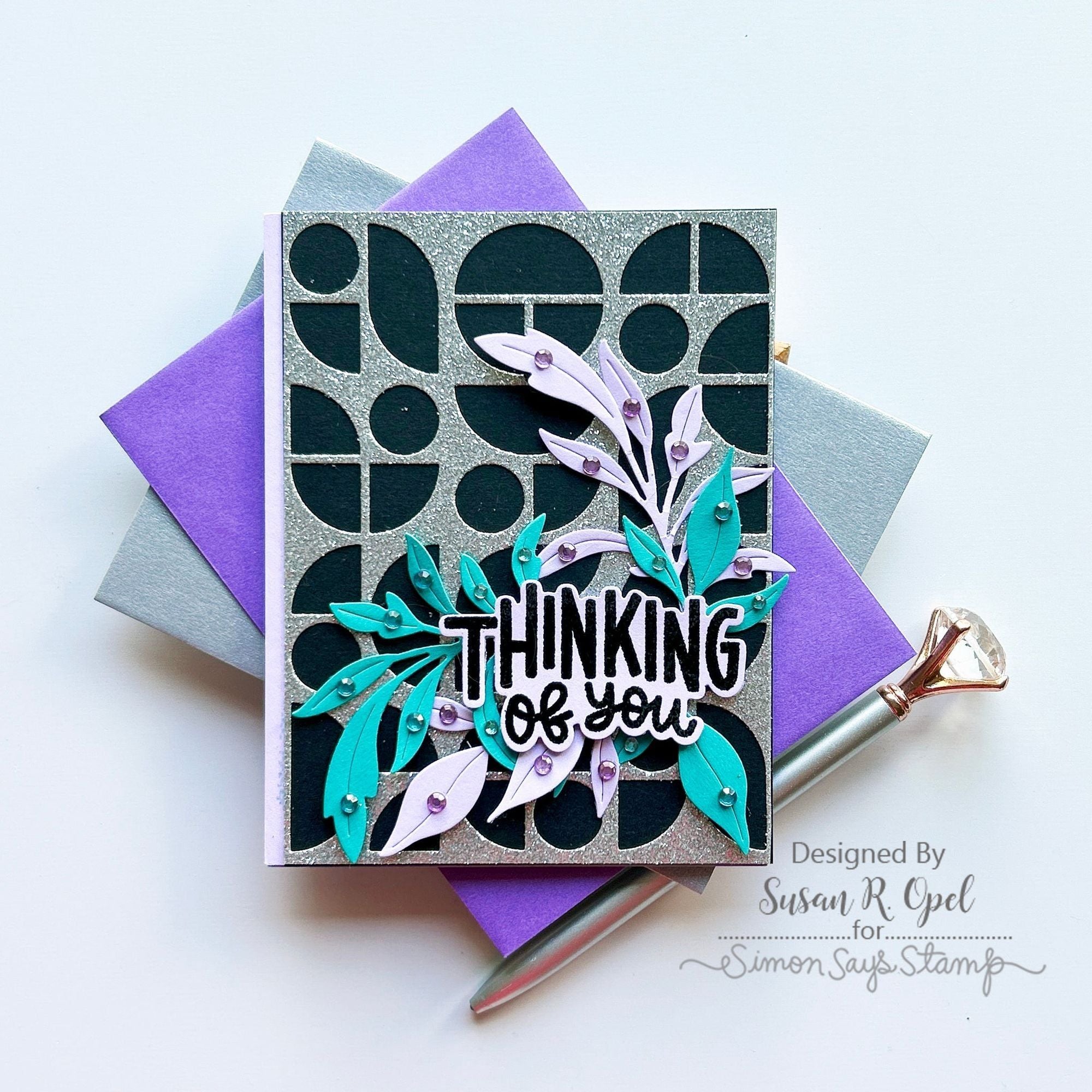The image showcases a beautifully designed greeting card and its accompanying elements on a white background. Central to the composition is the card, adorned with intricate cutouts and patterns. The topmost and most striking design features the black text "Thinking of You" in a layered cutout format, set against a silver, sparkly backdrop. Beneath this are delicate cutouts of pale lavender and teal leaves, embellished with amethyst and teal gems, respectively. These sit atop a series of geometric shapes composed of semi-circles and other forms that create an engaging and unique design.

The card is placed among two envelopes: a purplish one directly below it and a gray-silver one at the very bottom. These items cast subtle shadows on the white background, adding depth to the image. To the side of the card and envelopes lies an ornate pen, characterized by its large, jewel-like top which resembles a diamond, adding a touch of elegance.

In the bottom right corner of the card is the text, "Designed by Susan R. Opel for Simon Says Stamp."